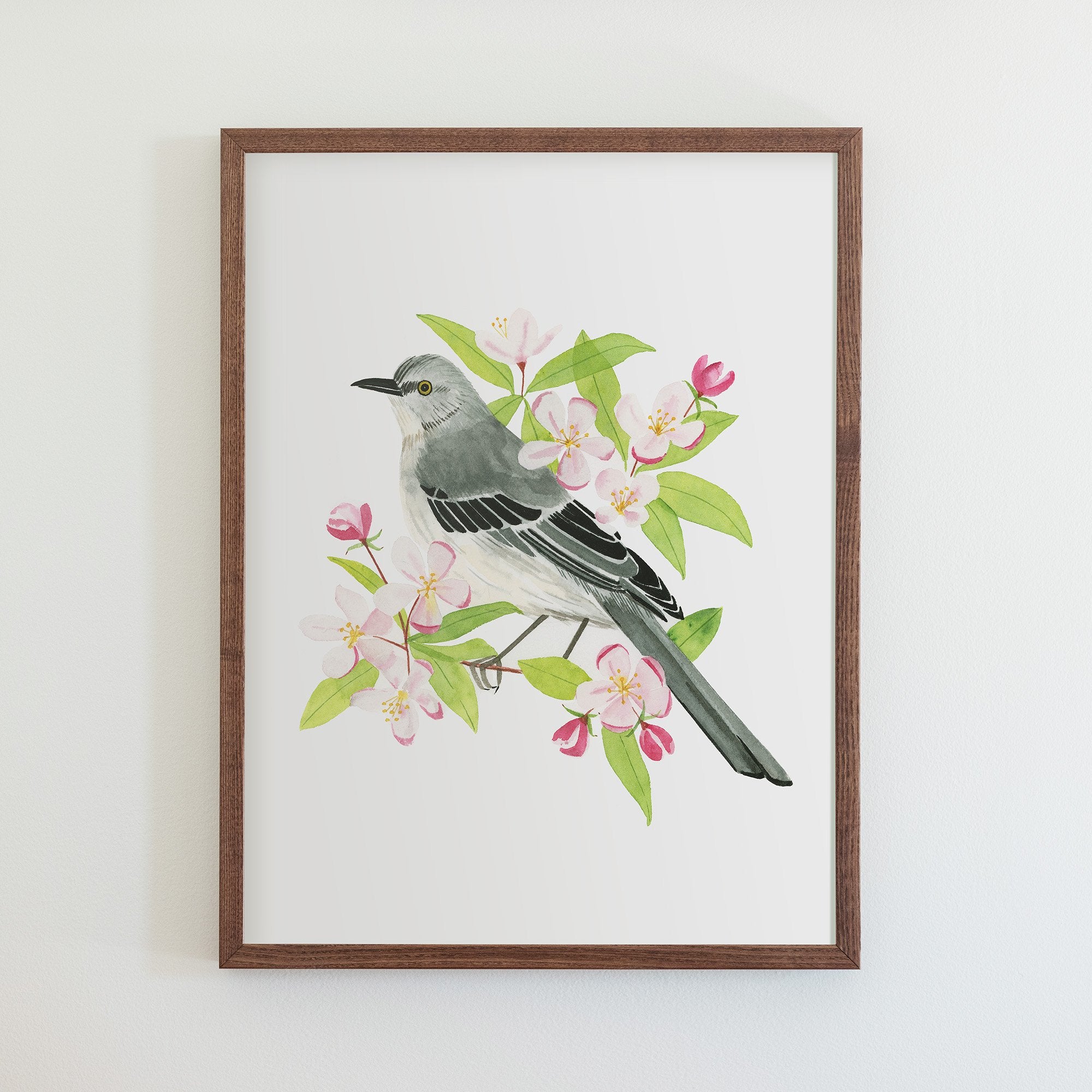This image features a detailed watercolor painting of a Northern mockingbird perched on a branch adorned with delicate apple blossoms. The artwork is set against a white background and is encased in a rustic brown wooden frame, mounted on a pristine white wall. The bird, facing left, showcases a striking plumage with a gray head, gray back, and black wings accented with some gray feathers. It also sports a long, pointed black beak and a gray tail, with distinctive white breast feathers extending up to its throat and a patch of black around its eyes and atop its head. The branch it perches on is adorned with blossoms that start as light pink and deepen to dark pink as they open, complemented by green leaves, characteristic of an apple tree. This beautifully captures the essence of the Northern mockingbird in its natural setting.